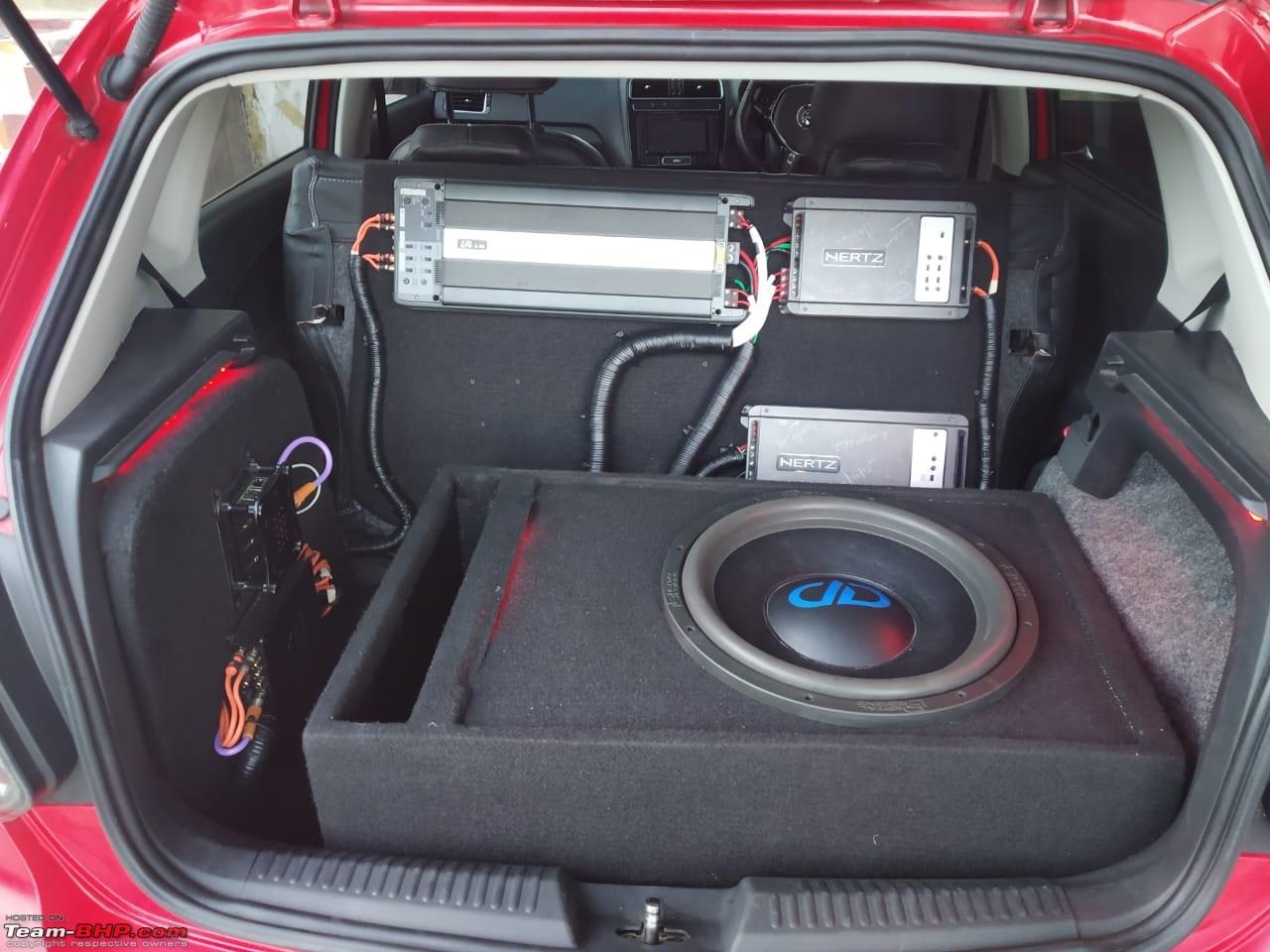The image depicts the exposed cargo area of a bright cherry red hatchback or small SUV, where the hatch is open, revealing a sophisticated car audio setup. Dominating the scene is a large black rectangular speaker box with a prominent round speaker, featuring blue lettering that is partially legible. The speaker box is encased in a black carpeted enclosure, which serves to amplify and protect the sound output. Adjacent to the speaker are several amplifiers, mostly silver in color and densely wired with cables of various colors, including green, red, orange, and purple. One of the components features the brand name "NERTZ" prominently. Additionally, in the bottom left-hand corner, the text "team-bhp.com" is visible in white and red. The exterior edges of the car are slightly visible, emphasizing the rich cherry red color, but no occupants are present in the vehicle. The overall focus of the image is on the detailed and elaborate stereo system set up in the vehicle's trunk.